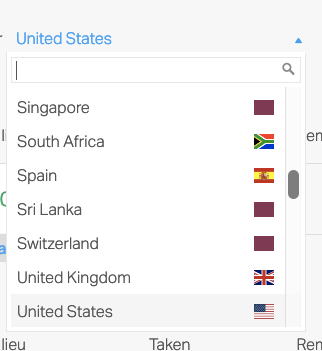The image displays a small pop-up window overlaid on a web page background, which is unreadable due to the pop-up's size. The pop-up window itself is white and features the text "United States" in large, bold blue lettering at the top left, alongside a blue triangular up arrow. Below this header, there is a rectangular text area with a gray cursor line on the left and a gray magnifying glass icon on the right, indicating a search or input field. 

Below the text area, the window lists several countries paired with their respective flags to the right. The first listing is "Singapore," accompanied by its red and white flag. The next is "South Africa," which has a flag featuring black, green, red, and blue colors. "Spain" follows, with a yellow and red flag. "Sri Lanka" is listed next, showing a solid red or brownish burgundy colored flag. "Switzerland" also appears with the same red burgundy flag, indicating this might be a placeholder image for missing flags. 

Further down, the "United Kingdom" is listed with its recognizable red, white, and blue Union Jack flag, followed by the "United States," also displaying its red, white, and blue flag. At the very bottom of the window, fragments of text appear: "LIEU" in black on the left, "taken" in black in the center, and "REN" in black on the far right.